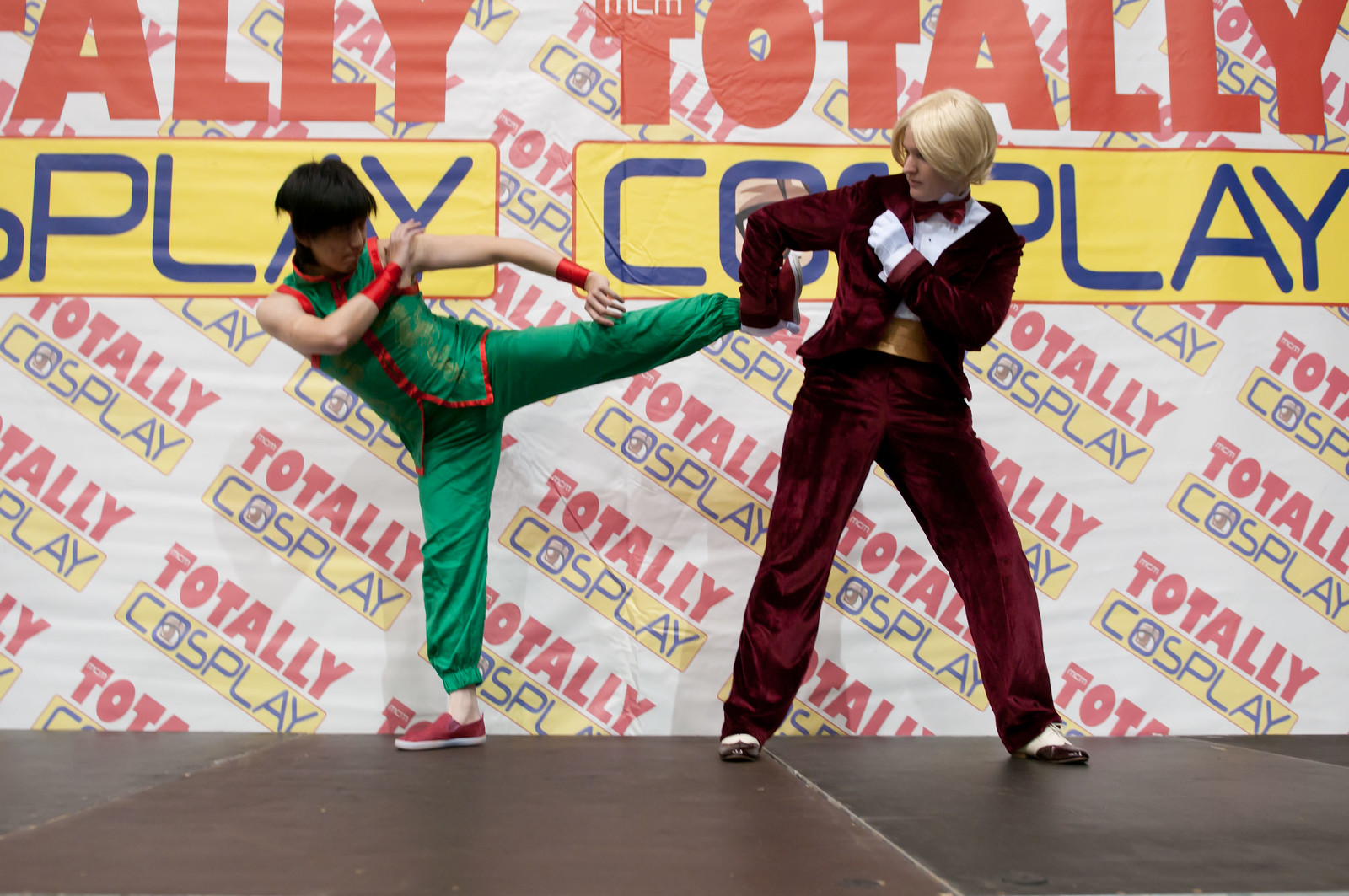The wide rectangular image captures two cosplayers engaging in a dynamic martial arts performance at the "Totally Cosplay" event, which is part of MCM in London. The floor at the bottom of the image, composed of long reddish-brown panels, leads the eye to the backdrop—a wall covered in the event's logo. The logo features the words "Totally" in bold red letters, and "Cosplay" in purple font on a yellow rectangle with an orange border, creatively incorporating an "I" in the "O."

On the left side of the image, an Asian male cosplayer in a bright green uniform with red trimmings and red slippers, performs an impressive kicking maneuver. His dark hair flows as he extends his left leg high, parallel to the ground. On the right, a blonde male cosplayer dressed in a burgundy velvet suit, complete with a bowtie, white shirt, and gold cummerbund, holds the green-clad cosplayer's leg, appearing to defend against the move. The action-packed scene unfolds on a black stage, with both participants embodying characters from a manga, surrounded by the vibrant branding of the "Totally Cosplay" event.